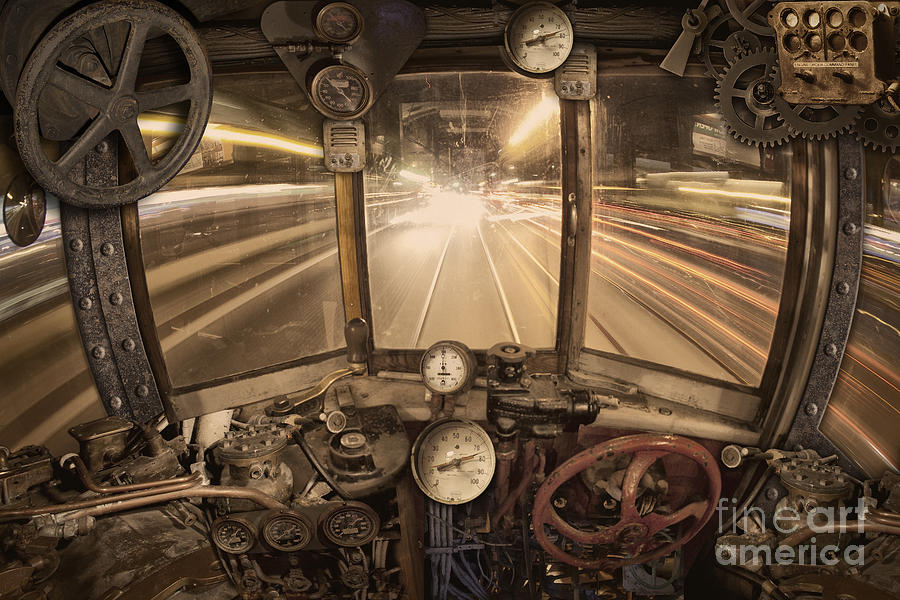This detailed image captures the interior of an old-fashioned, steampunk-styled train cab, brimming with a variety of metal mechanical parts and complex gauges. The central dashboard features numerous gauges, likely for monitoring vital metrics such as pressure or speed, with at least six to eight of them prominently displayed. To the right side of the image, a curious red steering wheel is visible, though it's unclear if it serves any actual steering function. The scene is awash with gears and assorted mechanisms, suggesting the intricate workings necessary to operate the train, which might be a steam train or a fantastical concept akin to one. Dominating the top right corner are additional gears, adding to the steampunk aesthetic. The view through the segmented windshield, which is divided into three parts, reveals a railway track extending out ahead. Above the main controls, a pull handle adds another layer of authenticity to the vintage design. A watermark in the lower right corner reads "Fine Art America," indicating this might be a conceptual artistic representation rather than a real photograph.